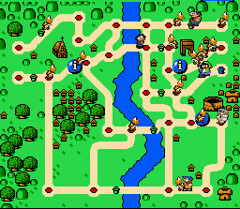The image is a still from an 8-bit style video game featuring an aerial view of a tan-colored maze or path spread across a square, grassy landscape. The background is a lighter green compared to the more vividly green, squat, bubble-shaped trees that are particularly concentrated on the left side. A blue river snakes vertically through the middle, diverting across the terrain. The path is interspersed with small red circles at intersections, likely indicating challenges or key points. The landscape is also dotted with small brown huts with peaked roofs. Scattered throughout the path are tiny characters navigating the maze, aiming to reach a final destination that appears to be either a castle or a water well, underscoring the game’s objective of overcoming these red-tinted obstacles along the way.